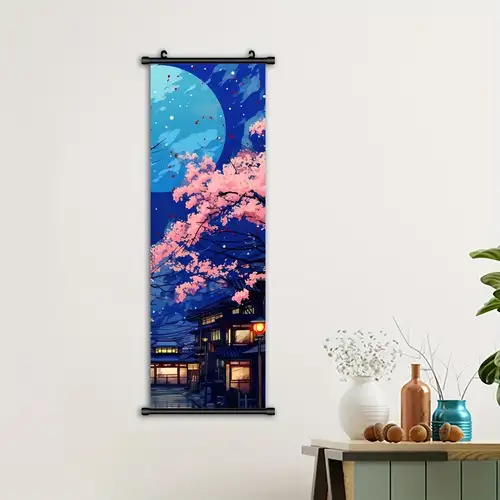The photograph captures the interior of a sparsely furnished apartment, highlighting an off-white wall adorned with a rectangular hanging. This decorative piece showcases a serene night scene featuring a royal blue sky with a pale blue moon, and the delicate branches of a pink cherry tree extending from the right side. At the center, the tranquil setting includes two buildings of classical Japanese architecture, characterized by their pagoda-style roofs and warmly glowing windows. In the bottom right corner of the image, a small table with gray paneling and a light beige top supports various decorative items: a white vase with white stems and berries, a sealed brown bottle, a small blue can-style vase filled with twigs, and a scattering of acorns. A hint of a green plant is also visible, adding a touch of nature to the minimalist decor.